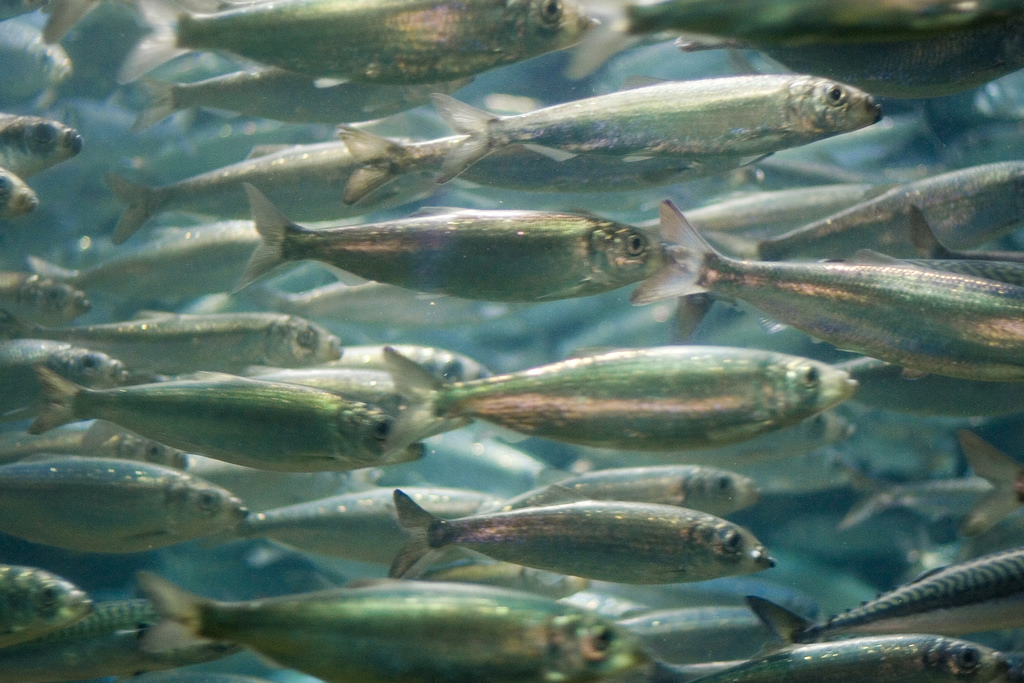This detailed wide rectangular photograph captures a mesmerizing underwater scene featuring a large, tightly-packed school of fish. Each fish, somewhat oval-shaped with pointed noses, is swimming uniformly towards the right. Their shiny, iridescent scales shimmer with a captivating mix of green, blue, and purple hues, accentuated by reflections of silver light. The fish possess tiny black beady eyes and distinctive lips, with the lower lip slightly wider than the upper. Their tails are comprised of two transparent gray triangular sections fanning out elegantly. The image, which appears to have been taken in a fish tank judging by the subtle, nearly imperceptible glare on the glass, shows a dense concentration of these fish in the foreground, while slightly blurred layers of additional fish recede into the murky, dark blue distance. This captivating scene, vividly blue and characteristic of an aquarium or museum display, underscores the serene beauty of the underwater world.